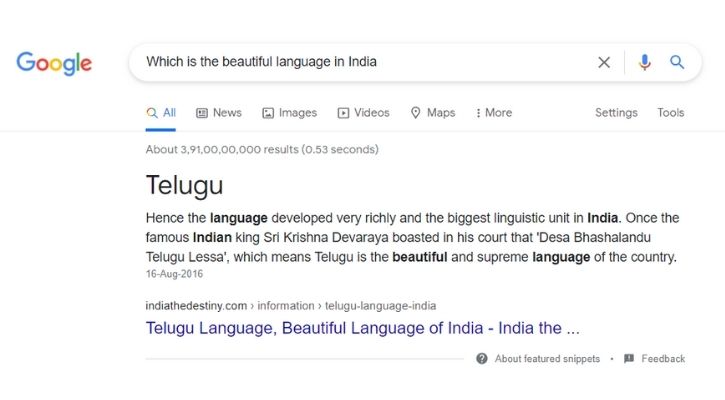The image is a screenshot of a Google search page featuring the traditional Google logo in the upper left corner and a search bar with the query: "Which is the beautiful language in India." The search bar also includes a gray 'X' on the far right, alongside a microphone icon and a magnifying glass symbol denoting search.

Directly below the search bar, navigation options such as "All," "News," "Images," "Videos," "Maps," and "More" are displayed, with additional settings and tools available further to the right. The search result prominently highlights the word "Telugu," spelled T-E-L-U-G-U, accompanied by information that states, "Hence the language developed very richly and is the biggest linguistic unit in India." 

The description continues, noting that the famous Indian King, Shri Krishna Devaraya, once proudly proclaimed in his court, "Deva Bhasha Landhu Telugu Lhasa," which translates to "Telugu is the beautiful and supreme language of the country." This information is dated August 16, 2016, and attributed to IndiaTheDestiny.com.

A clickable link titled "Telugu language beautiful language of India" is shown, pointing to further details on IndiaTheDestiny.com. Below the link, there are sections labeled "About featured snippets" and "Feedback."